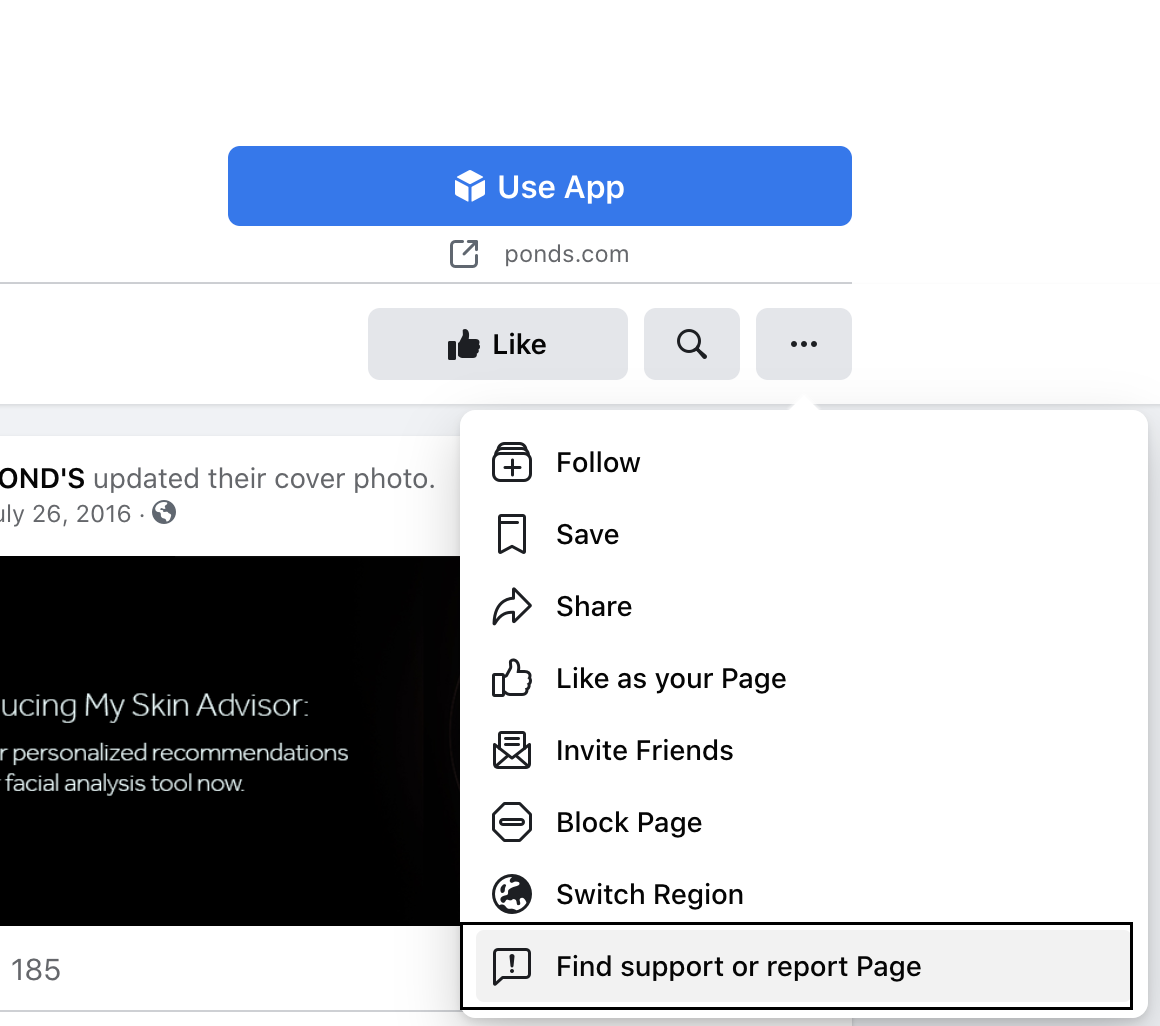The image appears to be a screenshot from Facebook. At the top, there's a blue bar with a 3D square icon. Directly below this, a square icon with an arrow pointing to the top right mentions "pons.com." 

The section in focus features typical social media elements such as a search bar and a three-dot menu, suggesting various interactions. Specifically, the options include "follow," "save," "share," "like," "invite friends," "block page," "switch region," "find support," and "report page." Additionally, there is an update notification that "Pons" has updated their cover photo.

Overall, this image showcases the user interface of Facebook, highlighting functionalities available for user interaction with a page named "Pons."